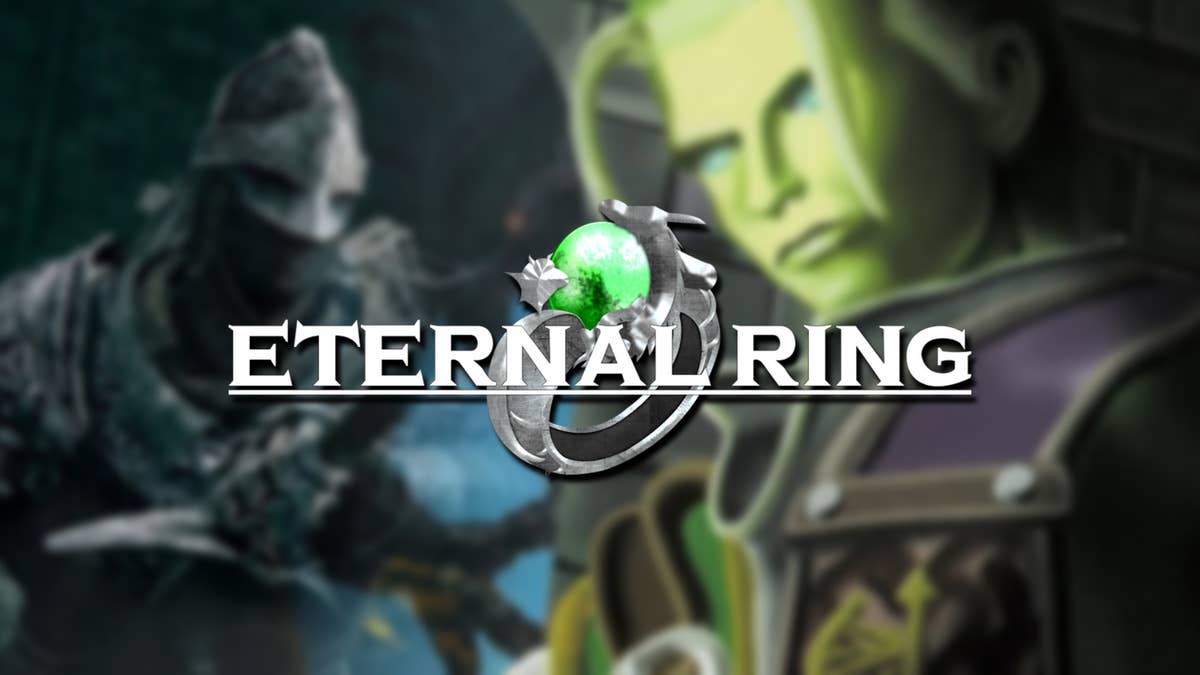The image is a horizontal color illustration designed as an advertisement banner for a game called "Eternal Ring". The bold, underlined title "ETERNAL RING" dominates the scene, with the word “Eternal” placed above and “Ring” below an intricately designed logo. The logo features a ring that appears to be a dragon wrapped around a spherical green gem, held in the dragon's mouth. 

In the blurred background, two animated characters are partially visible. On the left, a menacing figure with very white skin, bluish-gray areas around the eyes, and a scarf covering the lower half of his face stands in knight’s armor. This character seems to be eyeing the second figure suspiciously. To the right and slightly forward is a green-skinned character with elven features, light-colored hair, and blue eyes, clad in purple armor. This character appears to be fixated on the ring. The overall scene evokes a fantastical and competitive atmosphere typical for game advertisements.